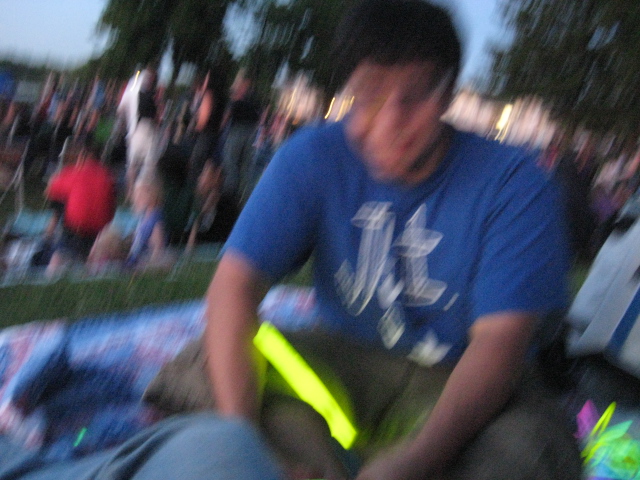In the center of this blurry image, a young boy sits on a blanket in a grassy field. He faces the camera, wearing a blue t-shirt and dark grey pants. His posture is slightly hunched as he sits cross-legged, with both hands positioned in front of him. The boy's medium-length black hair is visible, and he wears glasses. Between his crossed legs, a long, neon green light is noticeable. The background depicts a gathering of people, some standing and others sitting on blankets, with green trees framing the scene. The overall blur suggests that the image was taken in motion.